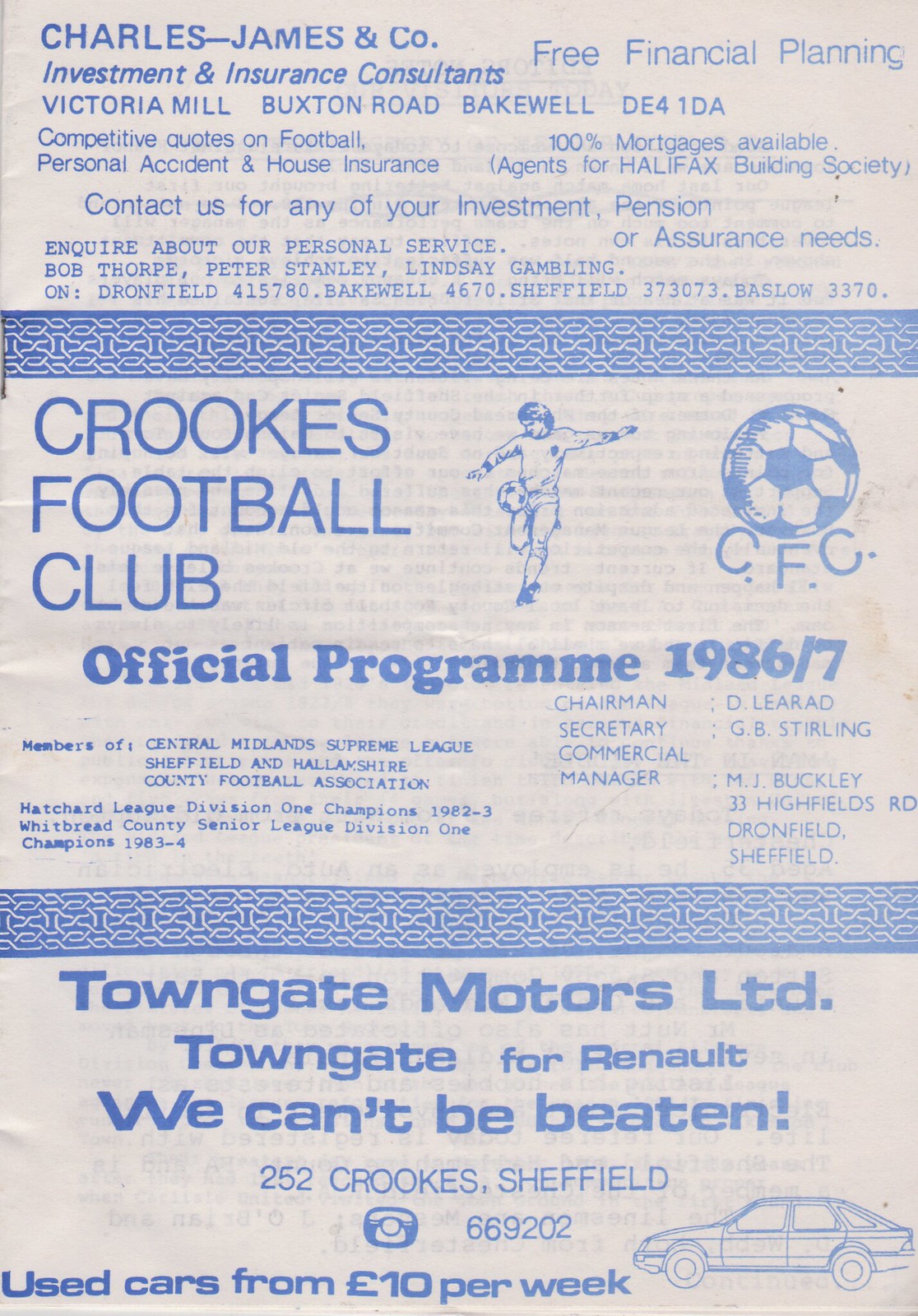This detailed poster or program cover primarily features blue lettering on a whitish-pinkish background, filled with a variety of information. At the top, the headline reads "Charles-James and Company, Investment and Insurance Consultants." Below this, it lists their location as "Victoria Mill, Buxton Road, Bakewell, DE41DA" and advertises "Free Financial Planning." The company offers "Competitive quotes on football, 100% mortgages available, personal accident and house insurance," and notes they are "agents for Halifax Building Society." It encourages readers to "Contact us for any of your investment, pension or insurance needs" and highlights a line about their "personal service" offered by Bob Thorpe, Peter Stanley, and Lindsay Gambling, with several contact numbers: Dronefield 415780, Bakewell 4670, Sheffield 373073, Baslow 3370.

Below this section is a wide blue stripe, followed by the announcement for “Crooks Football Club" in capital letters. To the right, there is an image of a soccer player with a soccer ball near their thigh, in mid-air. Alongside the player, another soccer ball is displayed with "CFC" underneath it. This part of the poster marks the "Official Program 1986-7."

Further down, after another wide blue border, is the advertisement for "Towngate Motors, LTD, Towngate for Renault." The slogan "We can't be beaten" is prominently displayed, along with the address "252 Crooks, Sheffield" and the offer of "Used cars from £10 per week." In the lower right corner of this section, there is a faint outline of a Renault car.